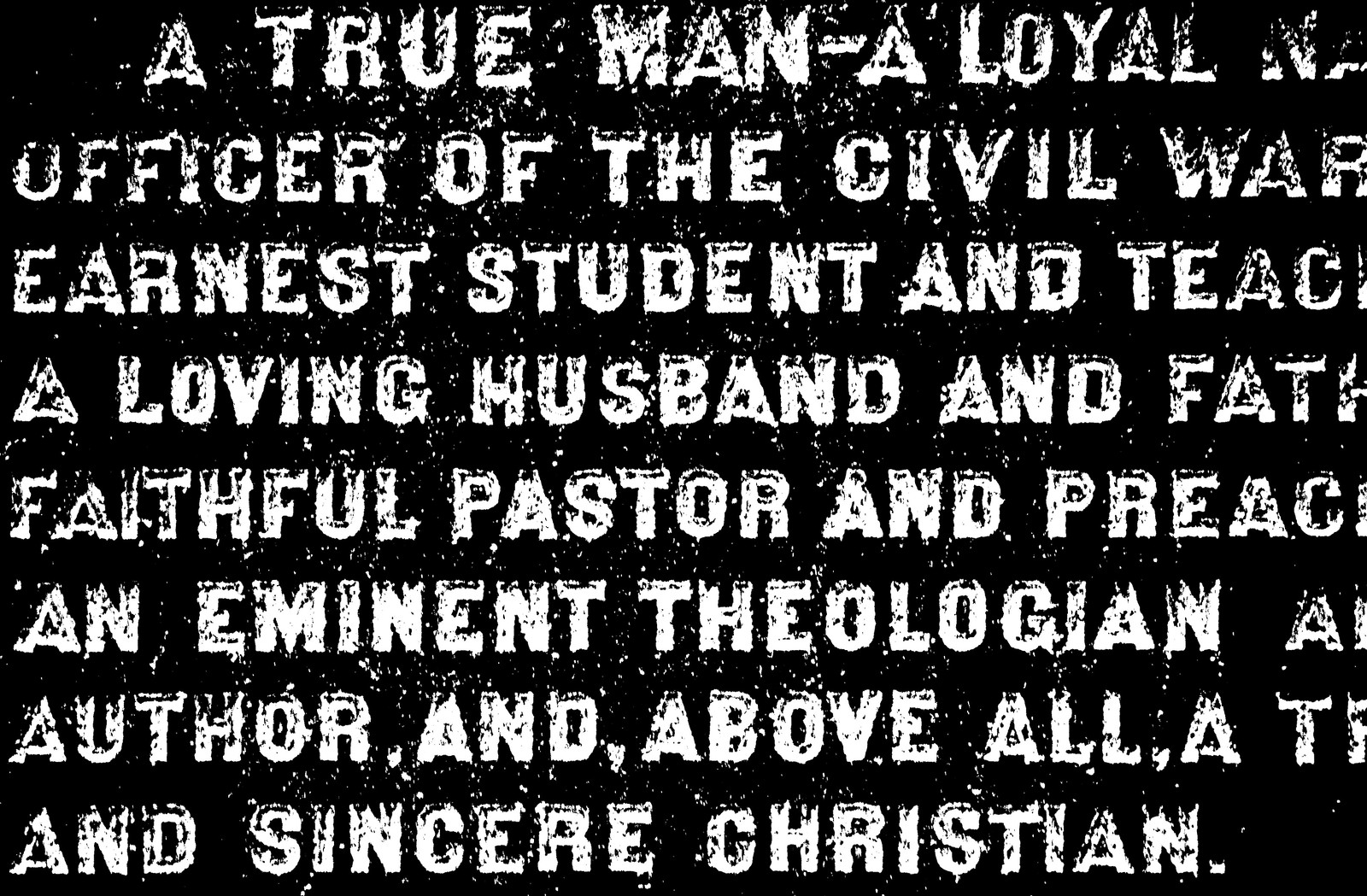This black-and-white image resembles a digital creation or potentially a photoshopped photograph of a gravestone, typically shared on social media. Displayed in white, gritty typography on a dark backdrop, the text reads: "A true man, a loyal officer of the Civil War, earnest student and teacher, a loving husband and father, faithful pastor and preacher, an eminent theologian and author, and above all, a sincere Christian." The worn and speckled appearance of the letters suggests imperfections akin to a malfunctioning printer, contributing to an overall impression of age and solemnity, echoing the gravestone's historic and eulogistic essence.